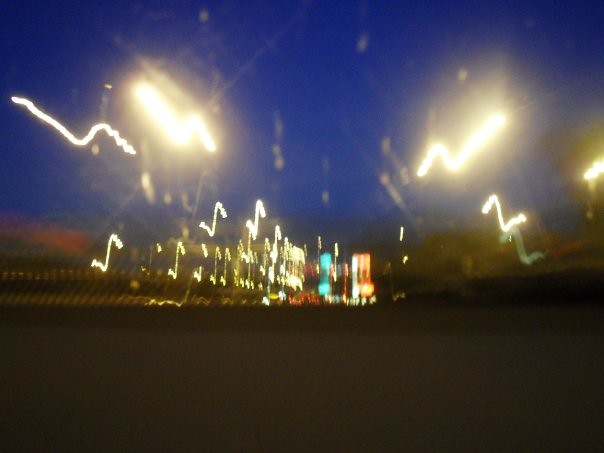This is a color photograph taken outdoors at night, capturing a blurry and dark street scene. The bottom third of the image is almost entirely black or dark gray, indicating that it might be a road or an obscured foreground. The top portion features a dark blue night sky, with two large, blurred light sources on either side, possibly street lamps, creating bright zigzag patterns against the sky due to the camera movement. Scattered throughout the middle section are numerous smaller, blurred lights, some appearing as reflections, suggesting that the photo might have been taken through a window. There are notable colors in the central area, including red, green, and white lines, which could represent distant vehicles or additional streetlights. To the left, there's a reddish and yellowish glow near the sky, likely from streetlights or the remnants of a sunset. The right side of the image hints at some foliage and a slight hill. The overall scene suggests an urban environment with blurred buildings in the background, illuminated by various orange, blue, and yellow lights that create a pattern of squiggly, indistinct lines throughout the photograph.